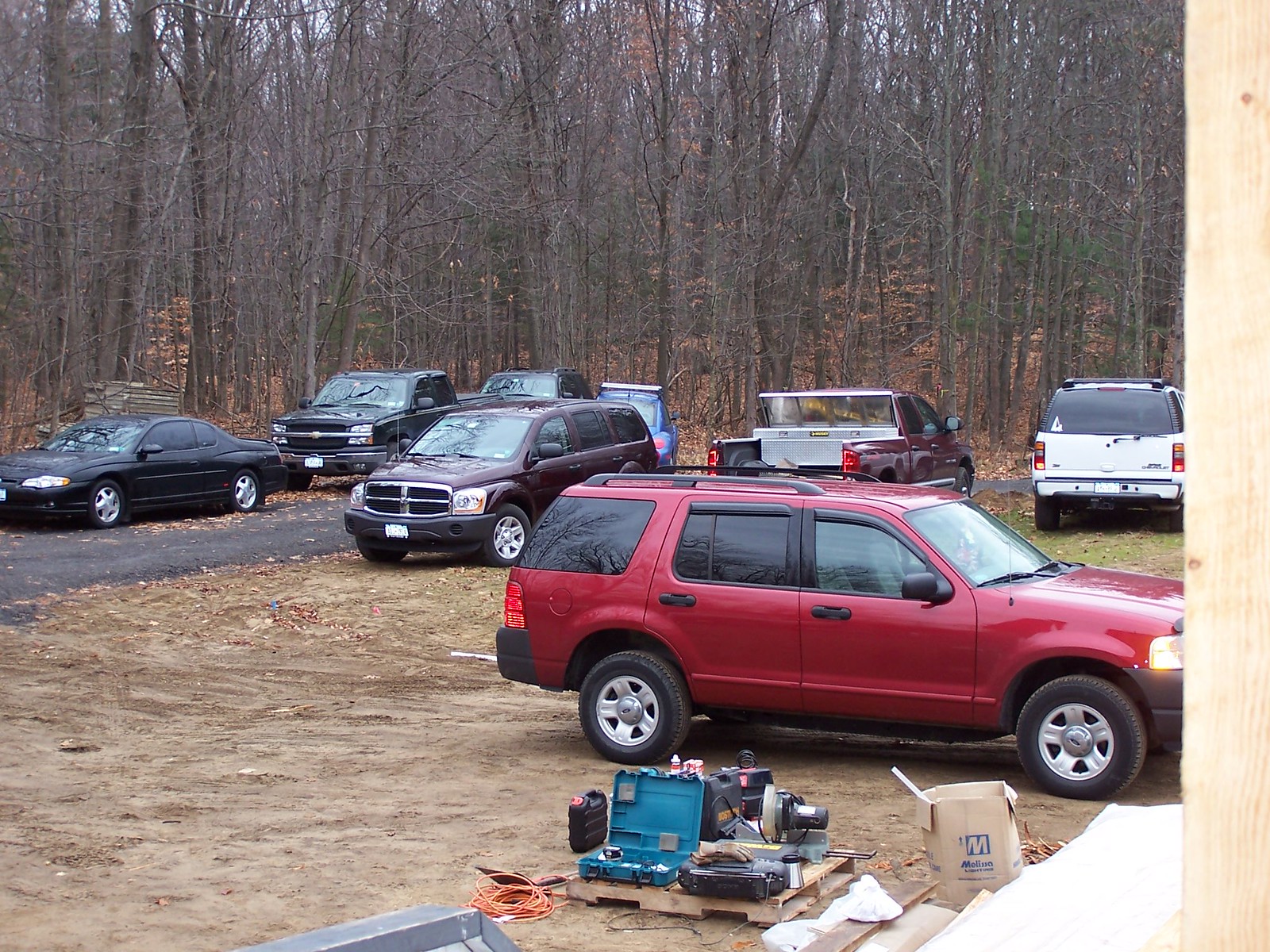The photograph, taken in the fall, captures a variety of vehicles parked on dirt ground in front of a wooded area with mostly leafless trees. In the background, two trees retain a few brown leaves, and a sliver of blue sky peeks through. Centrally, a burgundy SUV with three side windows and a sunroof is parked at an angle; its front points slightly to the left while the back angles right and away from the camera. Directly behind it is an indiscernible black car, partially visible, and to its right, a blue Volkswagen Beetle's rear end is seen. Further to the right, a burgundy truck with an open tailgate and a silver toolbox stands next to a white SUV with a large rear window. In the closer foreground, a road divides the scene, with more cars and trucks parked along its length. A notable feature near the road is a sideways parked burgundy car with visible headlights, taillights, and windows, accompanied by a small pallet of tools and an extension cord. The scene includes additional miscellaneous items, such as a drill case without the drill and a piece of new wood on the right, suggesting possible home renovation activities on a dead-end street.